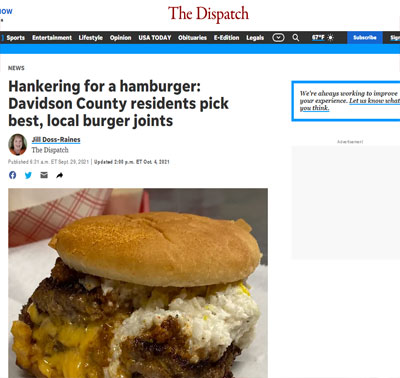The image depicts a screenshot of a webpage from "The Dispatch," prominently positioned in the center of the image. The word "now" is partially visible on the left side, but some text is cut off and unreadable. A black navigation bar below features various menu options: Sports, Entertainment, Lifestyle, Opinion, USA Today, Obituaries, E-Edition, and Legals. To the right of the navigation bar is a pull-down button whose function is unclear, next to a search button iconified by a magnifying glass symbol. It indicates the weather as 67 degrees Fahrenheit and sunny. Adjacent to it, a blue "Subscribe" button is visible.

The background is predominantly white, including the area beneath "The Dispatch," which is written in red text. Below the black navigation bar, a blue line stretches across, slightly differing in color from the other blue elements. Underneath, there's a section labeled "News" on a white background.

The headline, "Hankering for a hamburger, Davidson County residents pick the best local burger joints," is rendered in the largest black font. It is credited to Jill Doss Reigns, with her name underlined in blue. The article was published at an unspecified time (AM ET) on September 29, 2021.

A large picture of a hamburger, featuring a noticeable white component that is not clearly identifiable, accompanies the text, drawing significant attention as the main visual element.